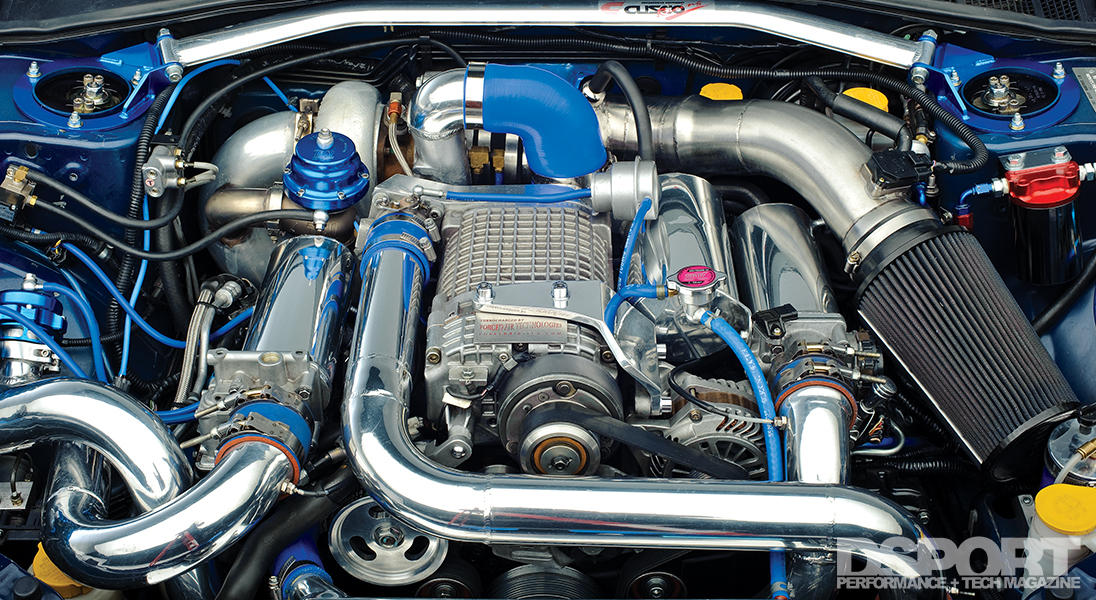The image captures a meticulously clean and brand new car engine viewed from under the hood. The engine features a sophisticated design with an array of blue-coated tubes intricately routed around the engine's perimeter, particularly concentrated on the left side. Prominent, gleaming stainless steel pipes dominate the center, so polished they reflect the surroundings. Red and yellow caps are scattered throughout, adding bursts of color among the predominantly metallic gray, blue, black, and yellow hues. A black belt is visible towards the upper right side, while the upper left houses blue compartments containing small objects, likely nuts and bolts. In the lower right-hand corner, there's a watermark that reads "DSPORT, Performance Plus Tech Magazine," indicating the source of the image. The entire scene is a high-resolution photograph emphasizing the state-of-the-art craftsmanship of the car's inner workings.